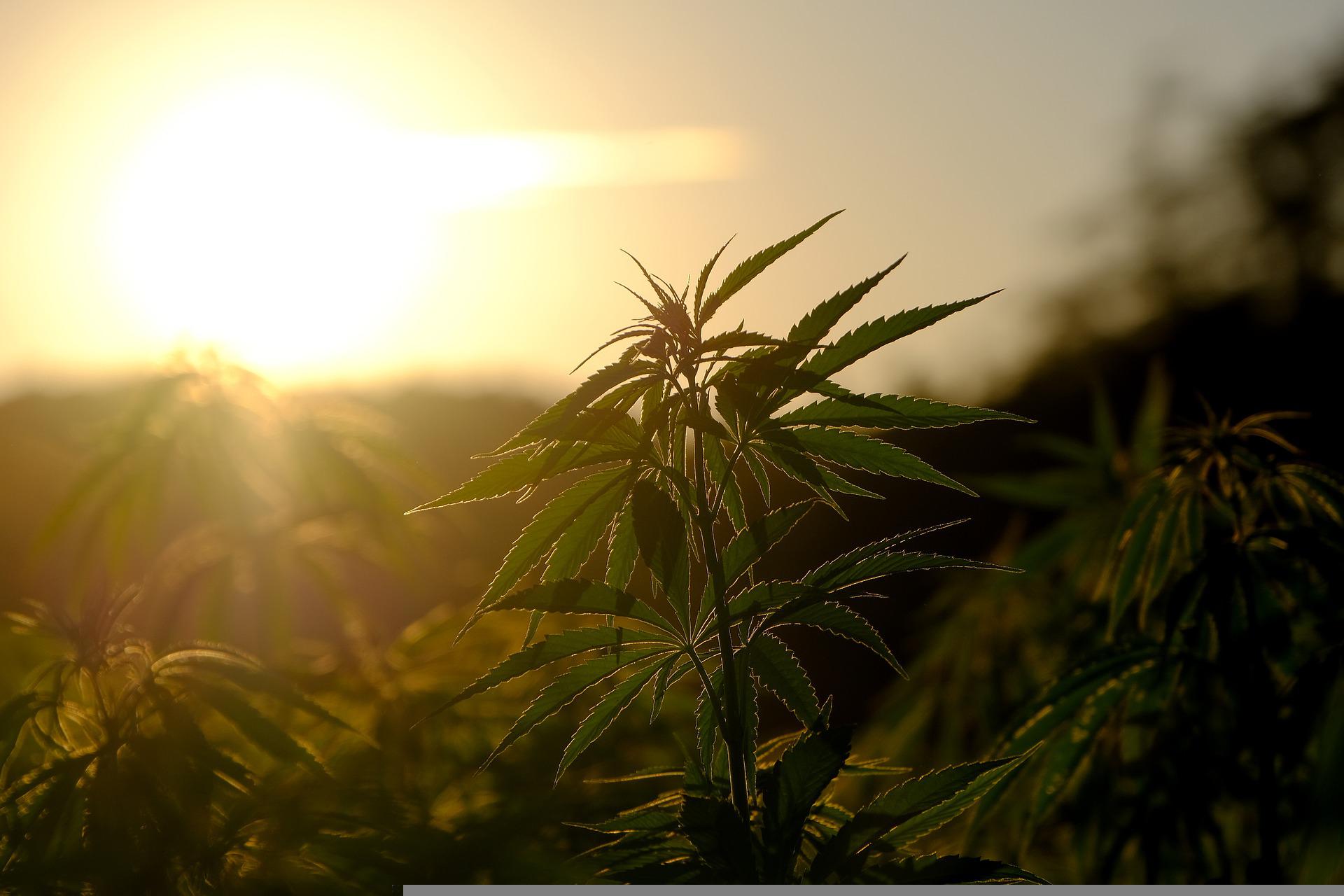This detailed photograph captures a close-up view of a lush green marijuana plant growing in a field in the desert. The image was taken at dusk, with the setting sun casting a golden hue over the scene and lending the entire field a warm, dusky atmosphere. The foreground features a single marijuana plant in sharp focus, showcasing its characteristic jagged leaves and nascent buds. In the background, other plants fade into a blur, emphasizing the depth and breadth of the field while also highlighting the solitary plant in front. To the left, the out-of-focus glow of the setting sun creates a striking contrast against the silhouette of the plant, emphasizing its vibrant green color and healthy appearance. The sky occupies the only plant-free space in the image, enhancing the natural beauty and tranquility of this desert landscape at golden hour.